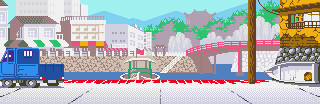In this detailed, digital rendering, likely from a video game, the scene captures the essence of a wharf by a river. To the left, a blue pickup truck with four grey wheels is positioned on a grey road near the water. Central to the image, a docked boat with green columns and a red flag appears, complemented by a rowboat in front of a long brown post. A striking red bridge, with white and brown undertones and red poles, stretches across the water in the background.

The foreground features a white wharf area bordered by rock walls leading up towards the bridge. A distinctive yellow and brown building is situated above these rock formations, accompanied by a brown pole and red linings near the blue water. The cityscape beyond includes numerous white buildings, some with distinctive green and white awnings, while another building boasts a red and orange covering. In the far background, the landscape is enriched by the silhouette of mountains and a scattering of green trees, creating a harmonious blend of urban and natural elements.